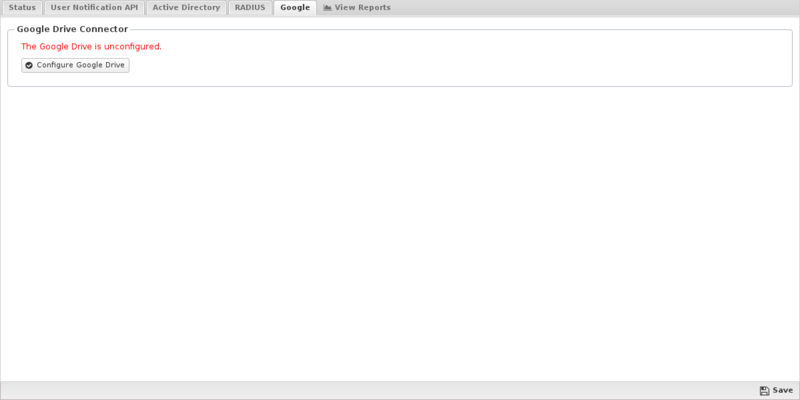This is a screenshot of a settings interface with a gray header bar running horizontally across the top. The header contains several categories on the left side: Status, User Notification, API, Active Directory, RADIUS (in all caps), Google, and View Reports. The Google category is currently selected.

Beneath the gray header, the background shifts to white. "Google Drive Connector" is prominently displayed at the top left, adjacent to a rectangular section that spans the width of the settings box. Within this rectangular section, "Google Drive Connector" remains anchored to the top left.

Inside this section, a message in red text indicates that the Google Drive is unconfigured. Directly below this message, a gray button labeled "Configure Google Drive" is positioned, featuring a check mark on its left side. The bottom-right corner of the rectangular section contains a "Save" button, completing the interface elements at view.